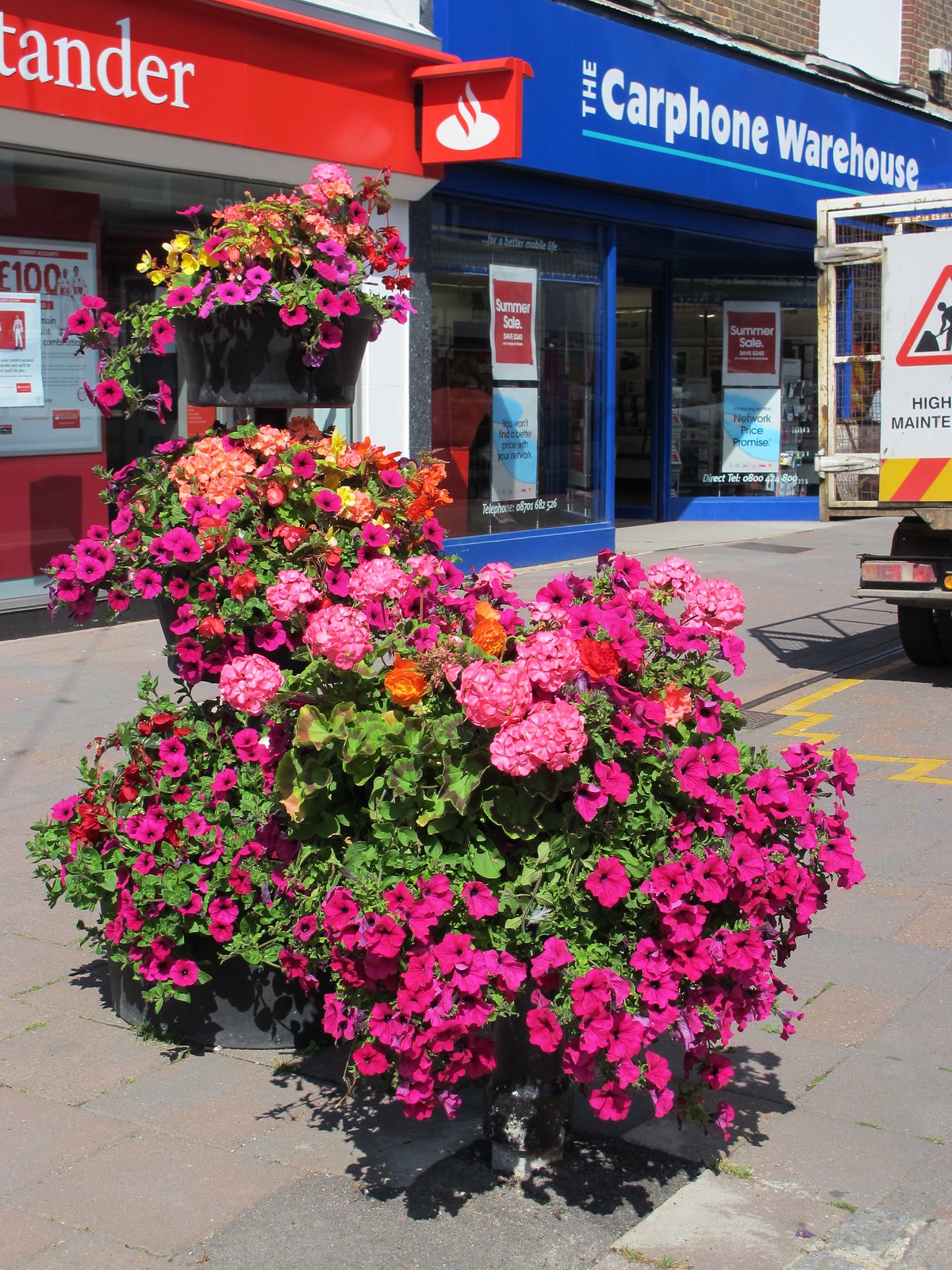The photograph captures a vibrant street corner bathed in sunlight, adorned with an array of colorful flowering plants situated in gray flower pots. Dominating the scene are vivid fuchsia, pink, dark purple, orange, and yellow blooms, predominantly appearing to be petunias, possibly of the vine wave variety. Additionally, there may be other types of flowers such as phlox, though they are harder to distinguish due to distance. These flowers overflow their containers, draping elegantly over the edges.

In the background, the image showcases the bustling facade of several businesses. To the right, a brick building features a striking blue sign with white lettering denoting "The Carphone Warehouse," accented by a lighter blue underline. Adjacent to it on the left, another establishment displays a prominent red sign with white letters, partially legible as "TANDOR". Both storefronts are adorned with additional signage in their windows.

Completing the urban tableau, a gray street runs past the corner where a truck is parked. The back of the truck prominently displays a caution symbol: a red triangle encapsulating a black icon of a person digging, against a backdrop of red and yellow stripes. This detailed scene not only highlights the floral beauty but also the vibrant commercial environment surrounding it.